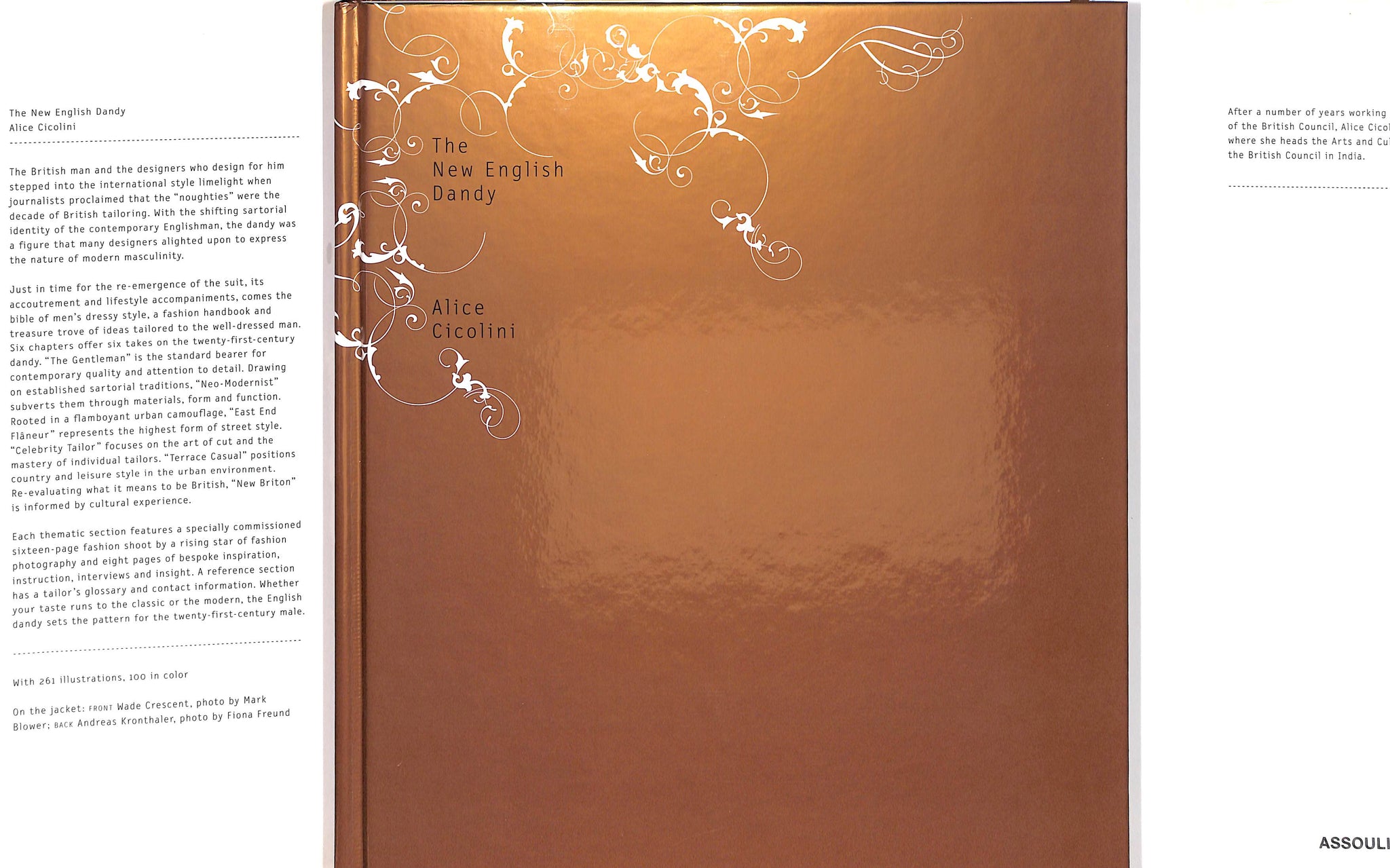The image showcases a book titled "The New English Dandy" by Alice Ciccolini, featuring a shiny brown cover with a reflective finish. The cover is adorned with intricate white line work in the upper left corner. The book rests against a plain white background. On the left side of the book, there's a detailed block of text describing the book, which includes a passage about the British man's evolution in fashion and how contemporary designers used the dandy figure to express modern masculinity. Additionally, the text reveals that the book contains 261 illustrations, including 100 in color, and mentions a jacket photo by Mark Blauer. On the bottom right corner, the publisher's name "ASSOULINE" is highlighted. The book’s thin structure is slightly evident from the shadow cast, adding depth to the image.